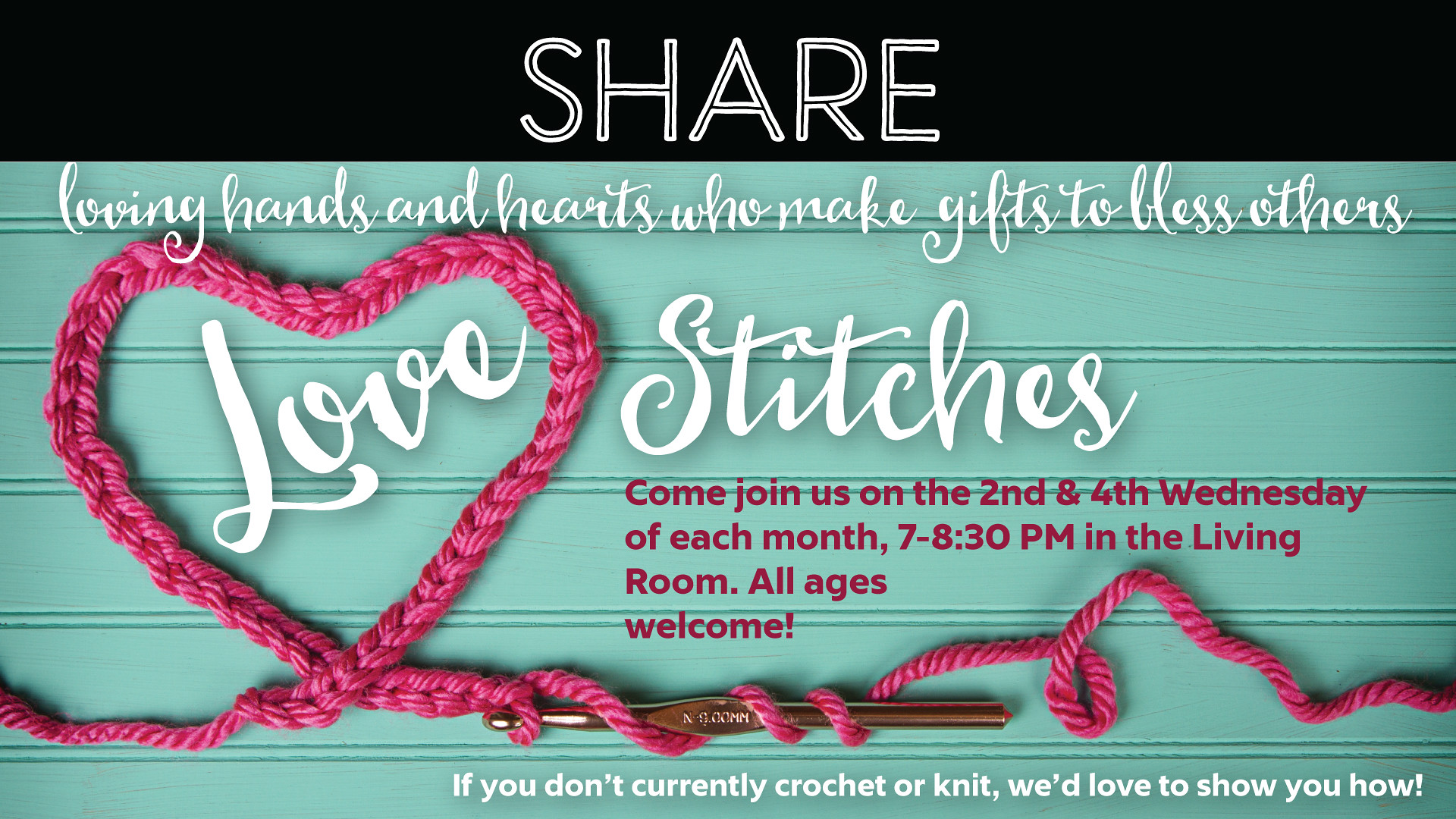The image is a detailed and colorful advertisement for a community knitting and crocheting event. At the top, a black band with bold white letters spells out "SHARE". Below that, the background is painted a teal blue, resembling horizontal wooden boards. To the left, a piece of pink yarn is shaped into a heart, still connected to a knitting needle, with the yarn trailing off to the right. Above the heart, in white letters, the text reads, "LOVING HANDS AND HEARTS WHO MAKE GIFTS TO BLESS OTHERS." Inside the heart, the word "LOVE" is prominently displayed, with the word "STITCHES" placed just outside of it. Further down, red text announces, "COME JOIN US ON THE SECOND AND FOURTH WEDNESDAY OF EACH MONTH, 7-8:30 PM IN THE LIVING ROOM, ALL AGES WELCOME." Lastly, at the bottom right corner in white text, it states, "IF YOU DON'T CURRENTLY CROCHET OR KNIT, WE'D LOVE TO SHOW YOU HOW." This inviting message encourages people of all ages to participate in creating heartfelt, handmade gifts while learning or sharing their skills in knitting and crocheting.